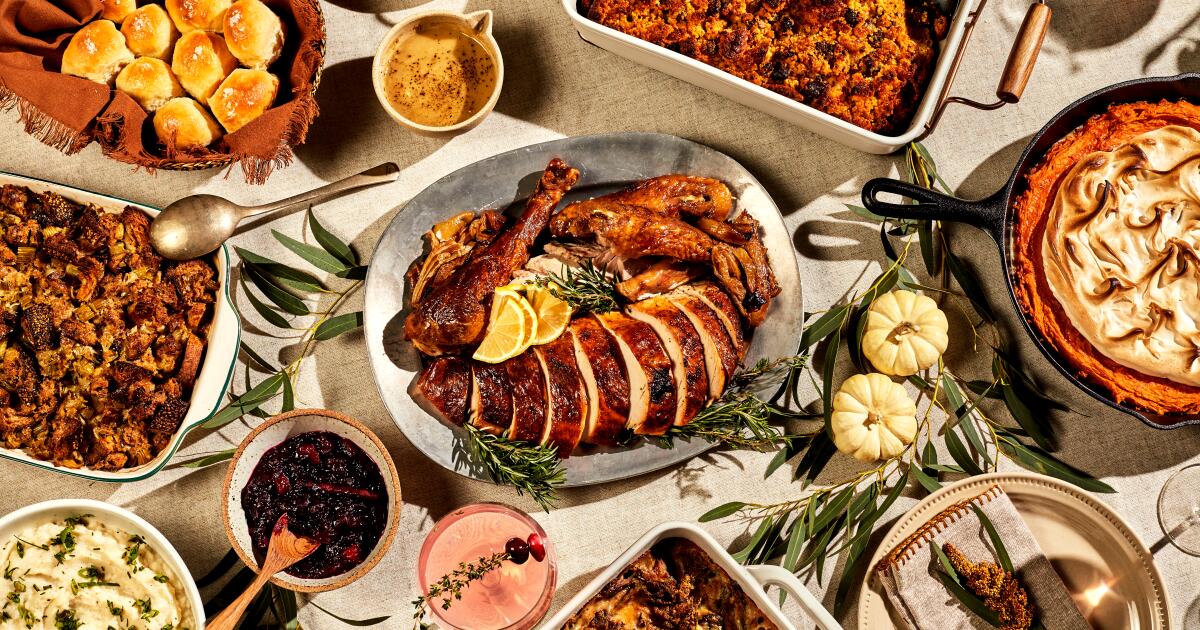The image depicts a lavish Thanksgiving meal spread across a table draped with a white tablecloth. At the center sits a silver oval platter showcasing a roasted turkey or chicken, beautifully sliced and adorned with oranges and green vegetables. Surrounding the bird, there are various side dishes: mashed potatoes on the bottom left, buns at the top left, a bowl of gravy above the buns, and two types of stuffing—one near the mashed potatoes and another near a sauce bowl to the right. Additionally, a black cast iron pan contains what appears to be a shepherd's pie with a distinguishing pie crust and mashed potato topping, positioned to the right of the central platter. Scattered across the table are small white pumpkins and green garnishes, enhancing the festive atmosphere. The overall feast also includes a wine glass and spoon, indicating a well-prepared and abundant meal.